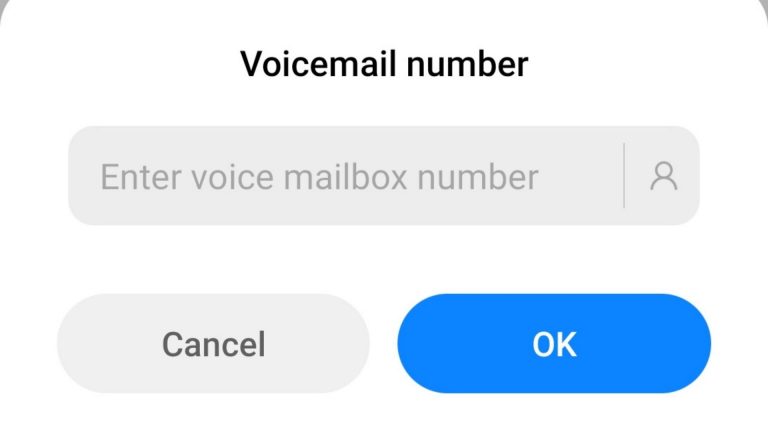This image depicts a user interface for a voicemail system. Centered at the top, black text indicates the voicemail number. Below this, a gray field prompts the user to "Enter Voicemail Box Number," presented in light gray text aligned to the left. Adjacent to the right of this prompt, separated by a vertical line divider, is a profile icon. Further down, two pill-shaped buttons are aligned horizontally; the left button is gray with the word "Cancel" in matching gray text, while the right button is blue with "OK" written in white. The entire layout is set against a clean white background, with the main elements centralized for a clear and straightforward user experience.